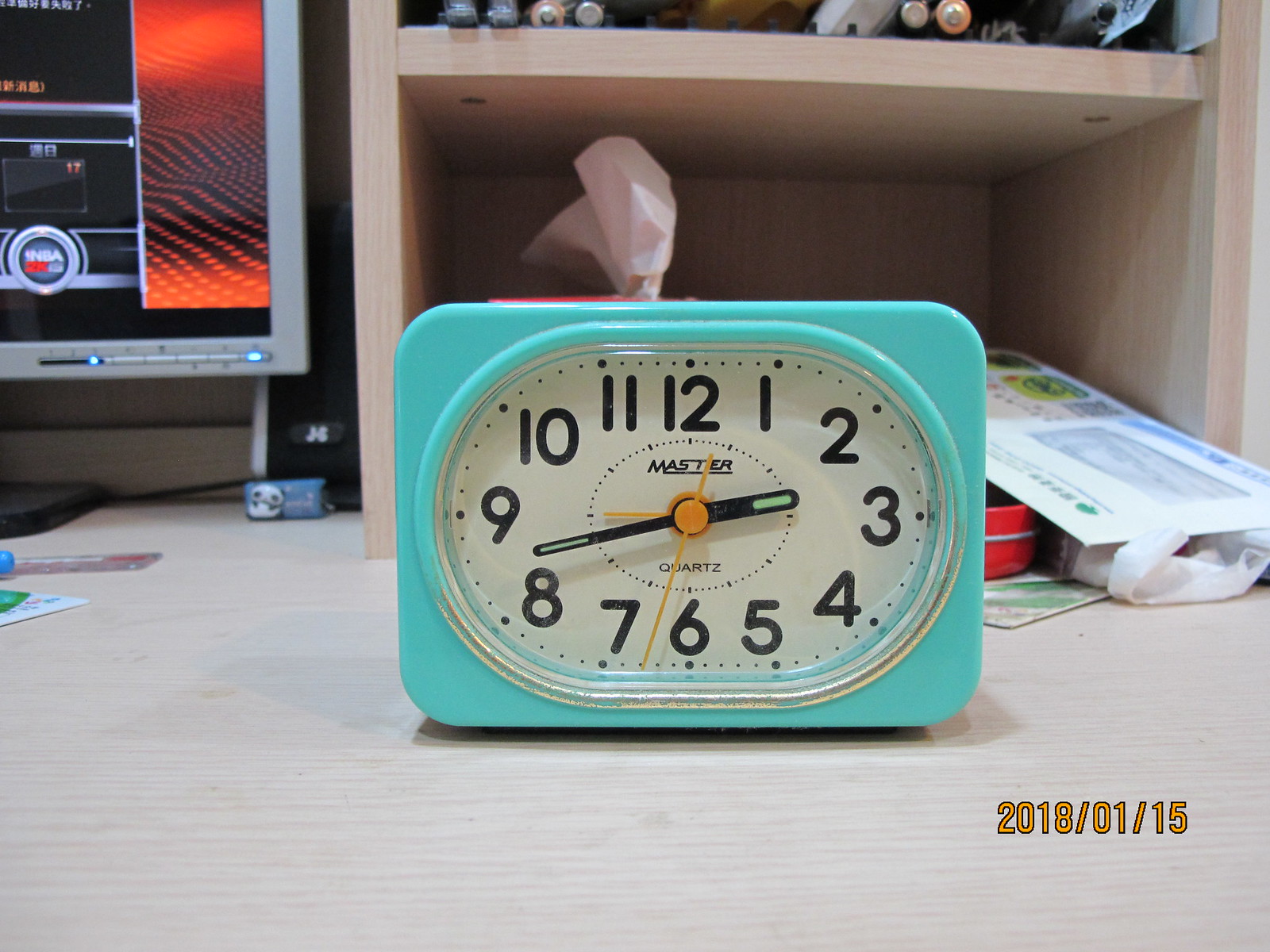This photo depicts a blue plastic square clock with an oval-shaped face dominating the center. The clock features large black numbers prominently displayed around its circumference and a smaller inner oval that bears the inscription "Master Quartz." The clock's hands are distinctive: a small black hour hand and a slender black minute hand, both adorned with tiny green lines in the middle, and a bright orange second hand. 

Positioned on a light-colored wood desk, the clock is accompanied by a backdrop of a computer desk setting. In the lower right corner of the image, there is a yellow digital date stamp reading "2018/01/15." Behind the clock, a shelf holds various items including a box of tissues, some mail, and a red tin container. A silver computer monitor appears on the left side of the image, displaying a black and orange interface with red accents, potentially featuring Japanese or Chinese characters. On the shelf above, a collection of cylindrical objects resembling batteries can be observed, alongside other small, unidentified items like a ruler, pencil, or eraser. The setting evokes a sense of an organized yet busy workspace.